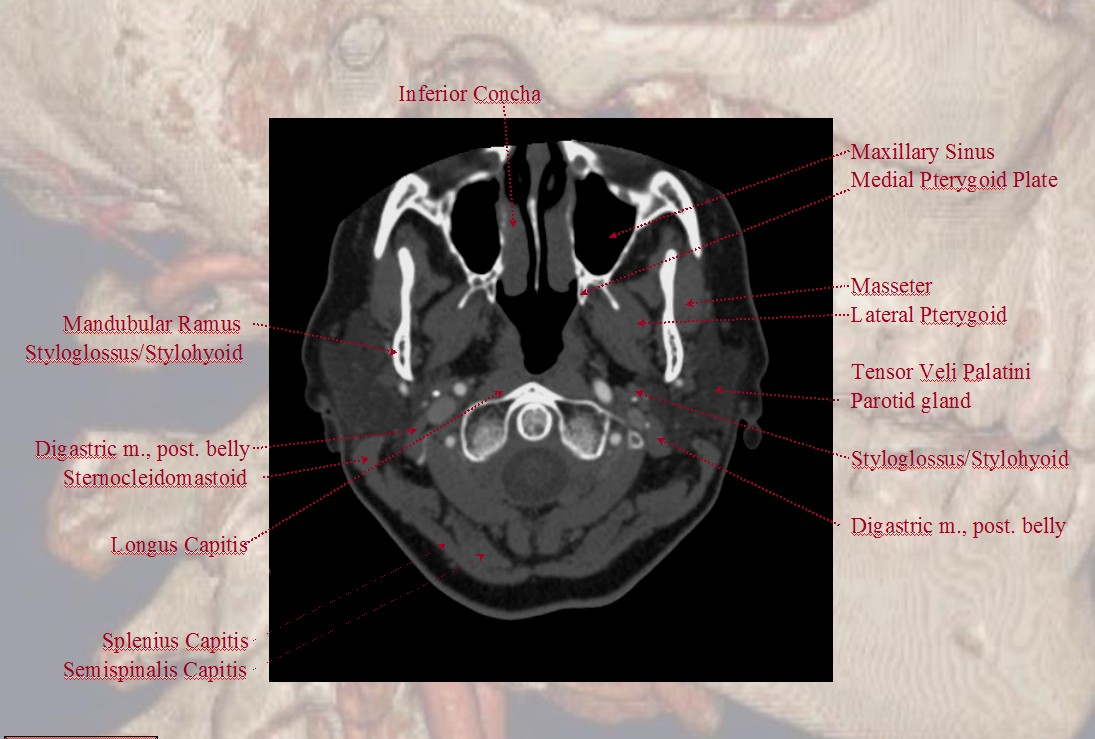The image is a highly detailed, medical instructional photograph showcasing a cross-section of the human skull and spinal column. Set against a black background, the central image resembles an x-ray and features various anatomical regions labeled with red text and arrows. These labels point towards key parts of the skull and neck, including the inferior concha, longus capitis, mandibular ramus, and lateral pterygoid. The square cut-out contains black-and-white representations of the skull's structure, with eyeball sockets near the top and the base of the head near the bottom. The background of the image depicts a close-up of the side of a skull, emphasizing the intricate bone structures. This detailed labeling is clearly intended for medical training, showcasing the precise anatomy of the skull and upper spine.